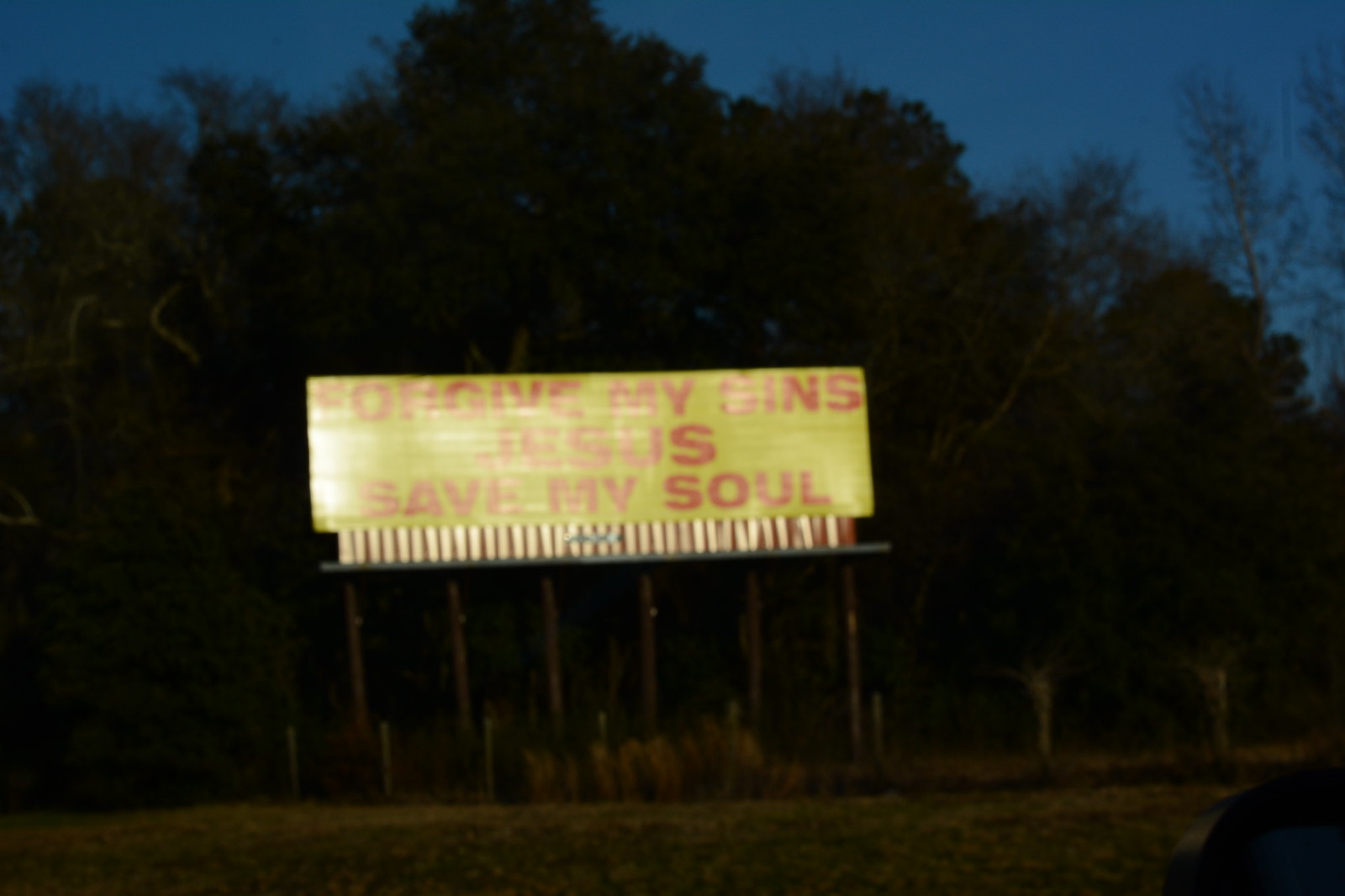The image captures a billboard prominently situated along the roadside, designed to convey a powerful message even to nighttime travelers. The billboard features a striking yellow background, with large, bold red capitalized text that reads, "FORGIVE MY SINS JESUS SAVE MY SOUL." The sign is illuminated by a few strategically placed lights, ensuring visibility of the message during both day and night. Due to the image being taken at night, the reflective glare from the lights on the billboard creates a bit of visual distortion, slightly obscuring the text. Behind the billboard, a dense, dark forest stretches into the background under a deep blue night sky. The overall scene is set against a serene yet somewhat mysterious backdrop, amplifying the solemnity and urgency of the message on the billboard.